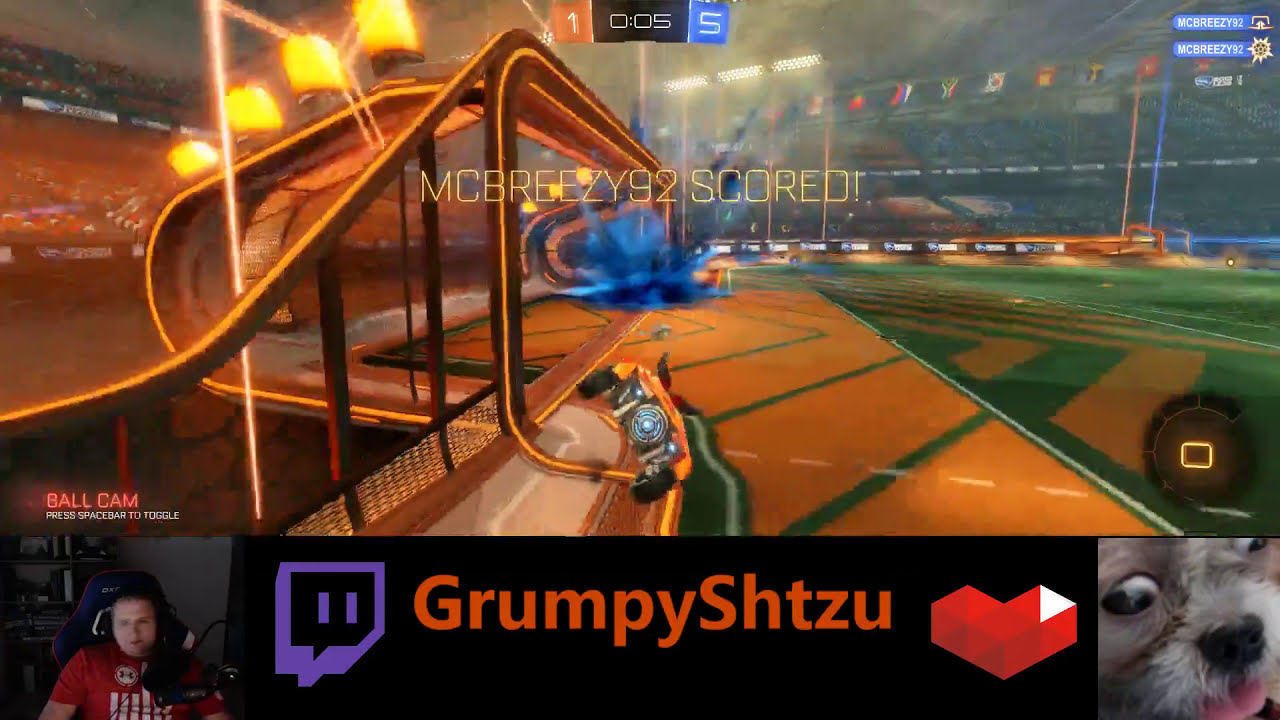The image is a detailed screenshot of a racing video game that incorporates elements of soccer, likely from a Twitch livestream. At the very top of the screenshot, a timer reads "0:05," with a scoreboard showing "1" surrounded by orange and "5" surrounded by blue. Below the timer and slightly to the right, there are two sections displaying the game players' names. From the upper right towards the center, a string of national flags is visible, adding a festive atmosphere. 

The game field is predominantly green with white stripes and patches of orange indicating the goal area. An open goal is visible on the left of a broad green field, adorned with orange highlights and surrounded by cheering crowds. A car in the game is seen balancing on its two side tires, moving towards the goal amid a black and blue puff of smoke, likely from an in-game effect.

At the bottom of the image, there is a rectangular strip containing a Twitch branding element with the text "Grumpy Shih Tzu" in the center, accompanied by a heart symbol on the right. To the left of this strip, a webcam feed shows a gamer wearing a red shirt with white vertical stripes sitting in a gaming chair, speaking into a professional microphone. On the right side of the strip, there is a close-up picture of a dog with white fur around its black nose and brown skin around its big, bright eyes, sticking its tongue out humorously.